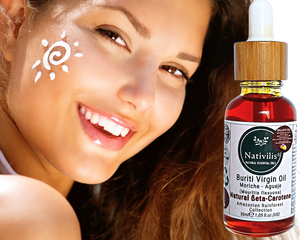This promotional image for Buriti Virgin Oil features a radiant young woman on the left and the product bottle on the right. The woman, with a glowing tan, long brown hair, and brown eyes, exudes a sense of health and happiness as she turns her beaming smile towards the camera. Her shiny lips are accentuated by pink lip gloss, and a cheerful sun graphic is painted on her right cheek. She also has her bare shoulder slightly visible to the left of the image, adding to the open and natural atmosphere.

The product itself, prominently displayed in a clear bottle with a brown cap, contains a reddish liquid. The white label with black and navy lettering identifies it as Buriti Virgin Oil, a natural source of beta carotene, known for boosting the immune system and offering various other health benefits. The label also features a dark green icon, typical of health products. The overall image has a clean, professional look, ideal for use on an e-commerce website.